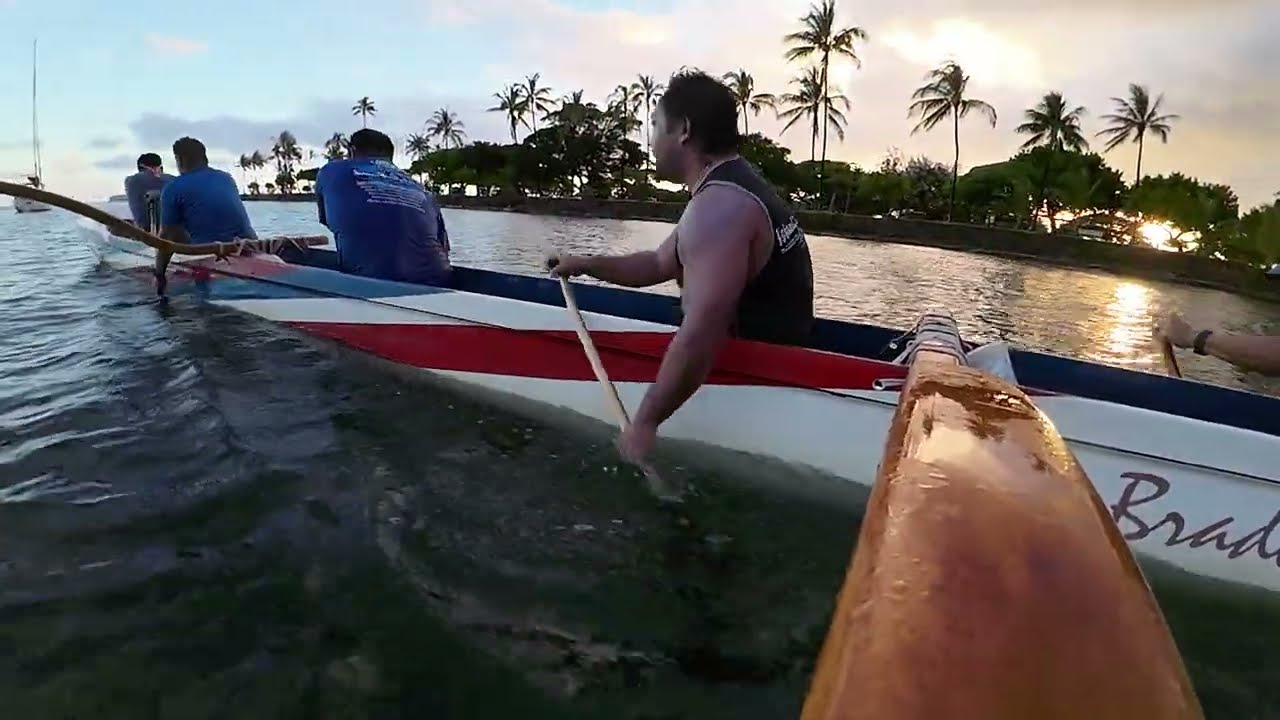A photograph depicts an action-filled scene of a narrow, white rowboat with red and blue stripes, marked with the partially visible script "B-R-A-D." The boat is populated by five rowers, with four clearly visible and the hand of the fifth noticeable. Three rowers sport blue t-shirts, while one, possibly of Samoan or Hawaiian descent, wears a black tank top and a necklace. This person, along with another rower, has their oar in the calm water, suggesting the boat is in motion. In the distance, a sailboat without its sail unfurled glides along, while the horizon showcases a tropical shoreline lined with tall palm trees. The sun sets behind the land, casting a warm glow over the serene scene, which is enhanced by the clear sky dotted with pretty clouds. The image seems to have been captured with a fisheye lens, possibly from a GoPro, providing a dynamic, slightly curved perspective of the tranquil tropical waterscape.